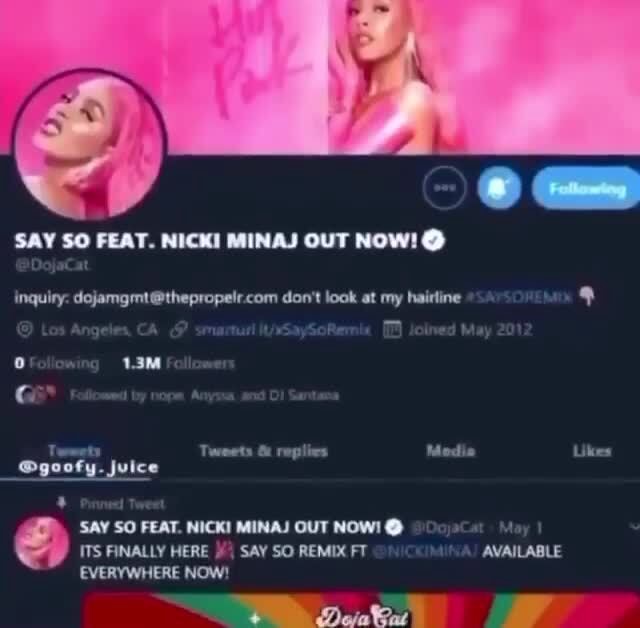The image is a square screenshot featuring a musical artist amid a vibrant, hot pink backdrop. Central to the image is Nicki Minaj, who faces the camera while wearing a pink glove. A circle frames her face, and the words "Say So featuring Nicki Minaj out now" in white text are prominently displayed below her. To the right, three icons include a follow button and the label "@Doja Cat." An inquiry web address is present beneath this information, alongside the phrase "Don't look at my hairline." The image notes that Doja Cat is from Los Angeles, California, and has 1.3 million followers, with her account joined in May 2012.

Below this information, the image lists some followers, followed by a menu at the bottom with tabs labeled "Tweets," "Tweets and replies," "Media," and "Links." A pinned tweet beneath this menu reads: "Say So featuring Nicki Minaj out now, it's finally here, say so remix featuring Nicki Minaj available everywhere now." The image's lower edge is cropped, but a rainbow-colored background with the text "Doja Cat" is partially visible.